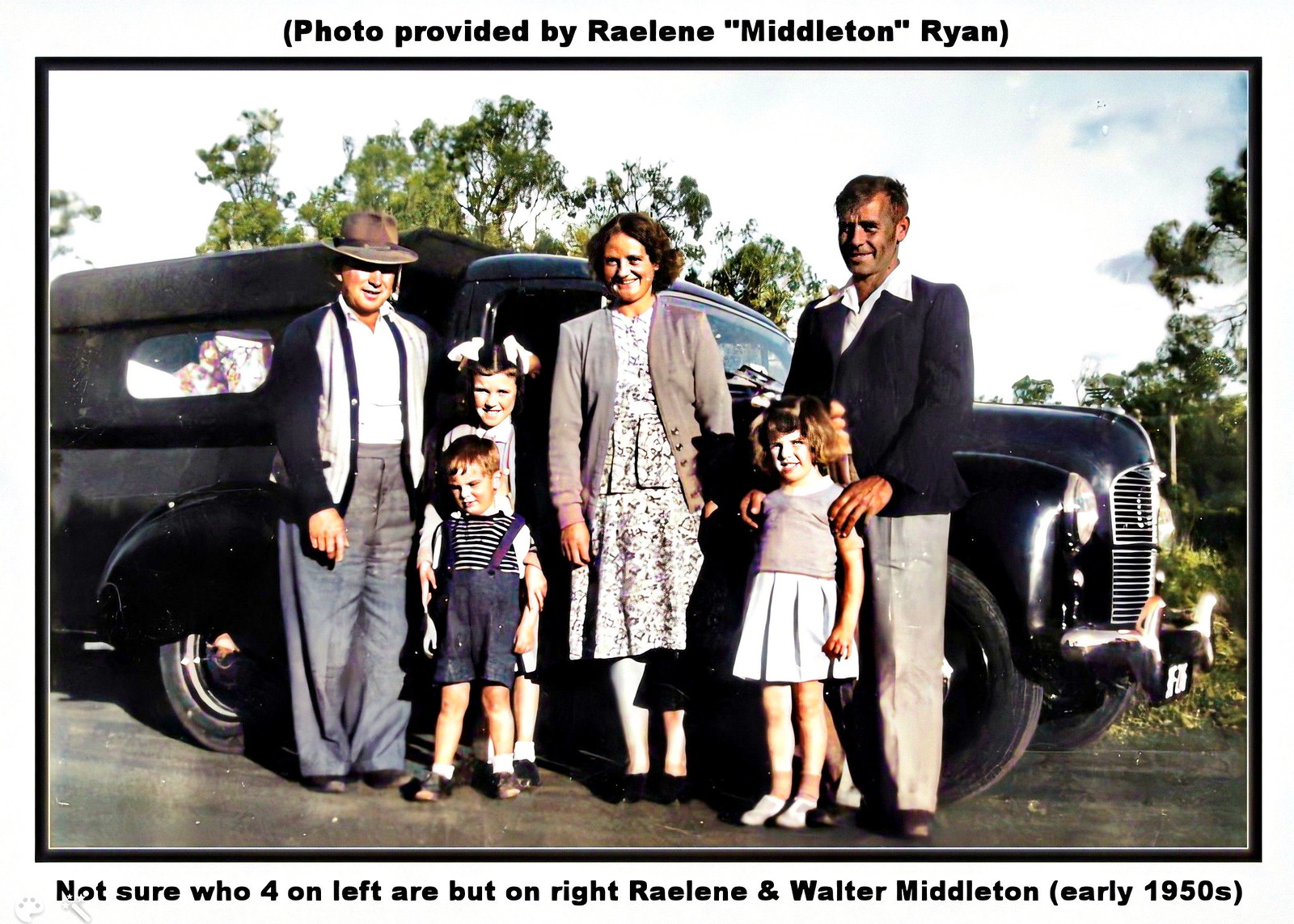This vintage photograph, provided by Raylene Middleton, depicts a family standing in front of a black 1950s truck, surrounded by a landscape of distant trees and an open sky. Arranged in a horizontal rectangle with a black outline, the image features six individuals, from left to right: an older gentleman in a brown hat, jacket, and gray pants, a girl with bows in her curly brown hair standing behind a young boy in blue and white striped overalls and sandals, a woman with short curly hair in a light-colored jacket and floral dress, a little girl in a purple top and white skirt, and finally, a man in a blue jacket and light gray pants with a white-collared shirt underneath. The woman and man on the right are identified as Raylene and Walter Middleton, captured in the early 1950s, as noted by the caption below the image. The photograph, originally black and white, has been colorized to enhance the nostalgic feel of the 1950s attire and setting.